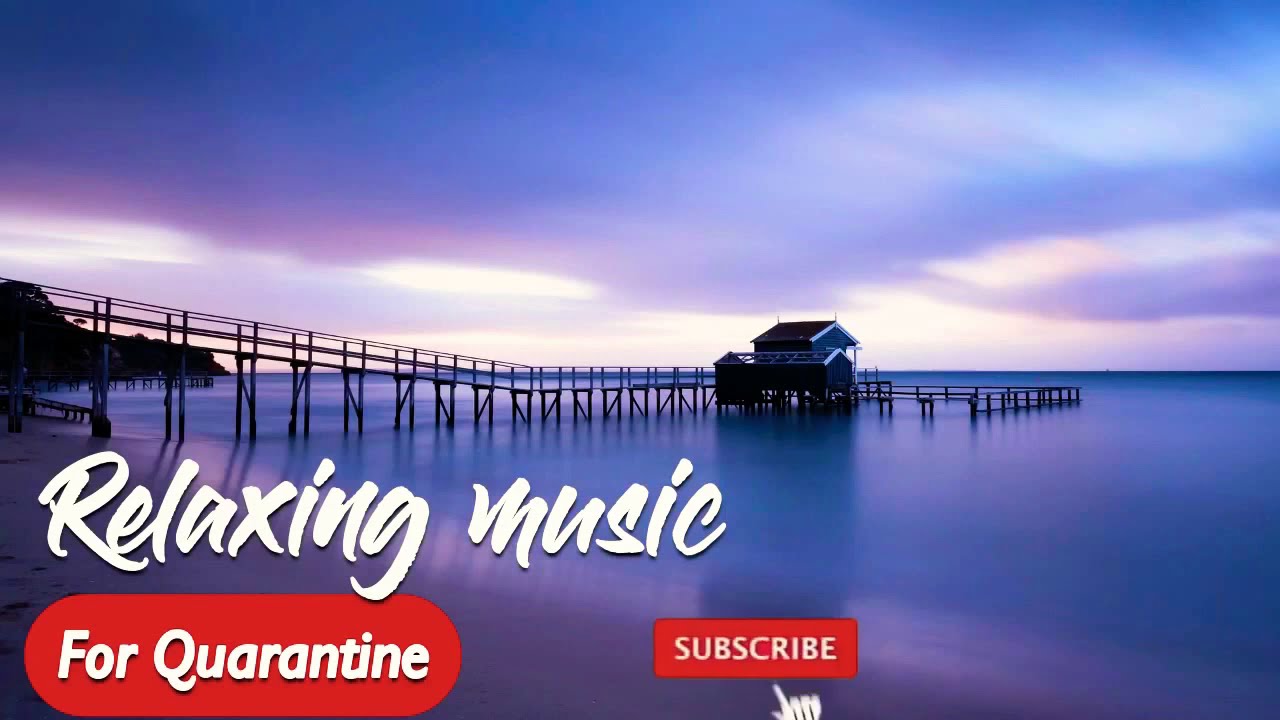The image depicts a tranquil scene of a large body of water, possibly a lake, reflecting the stunning hues of the twilight sky. The sky is adorned with partly cloudy conditions, radiating a blend of deep blues and pinkish purples, with the colors mirroring vividly on the water's surface below. A wooden dock extends diagonally from the left-hand side of the image, about 60% up, and shifts horizontally towards the right, forming an L-shape. At the center of the dock in the distance stands a small hut or boathouse with a triangular roof, offering a serene resting spot. Behind the dock, a small strip of land gently juts out, adding a subtle backdrop to the scene. In the lower-left corner of the image, bold white text reads, "Relaxing Music," accompanied by smaller text below stating, "For Quarantine." At the bottom center, there is a traditional red subscribe button with a hand-shaped cursor hovering over it, inviting viewers to engage. The entire image is bathed in a dreamy, almost purplish tint, suggestive of post-processing effects to enhance its calming aesthetic.